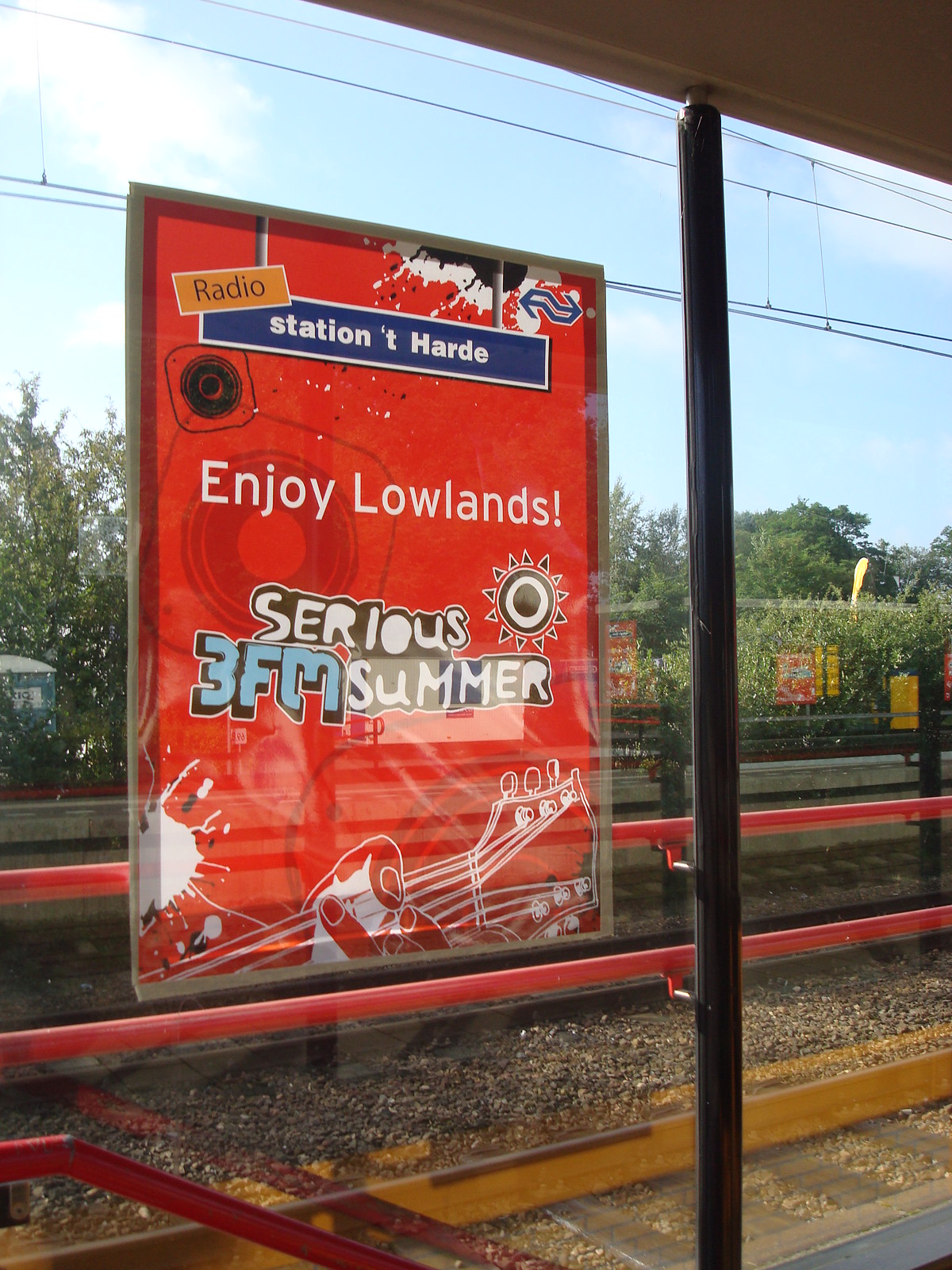This image captures a scene outside as viewed from within a building through a large, tall glass window, which is framed in silver. Prominently hanging on this window is a red poster for a radio station. The poster features a blue rectangular area at the top with white text that reads "Radio Station T. Hardy." Below this, it says "Enjoy Lowlands" and beneath that in more stylized text, "Serious 3FM Summer." Above the text, there is a black and white drawing of a sun with a white ring inside it, and at the bottom, a black and white sketch of a hand playing the neck of a guitar. Through the window, one can see several sets of train tracks and a boarding area for a train. Beyond the tracks, there's a landscape filled with tall green trees and greenery extending into the distance. The scene is bathed in daylight, evidenced by the blue sky with some white clouds. Additionally, power lines can be seen running high across the outdoor space.